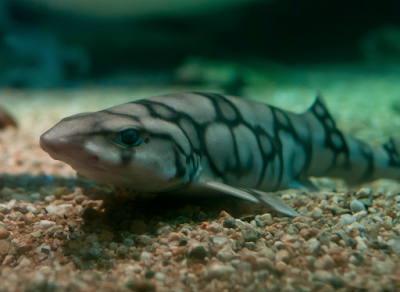In the image, a small fish rests on a bed of multi-colored gravel at the bottom of what appears to be an aquarium, although it could also be a natural underwater setting. The gravel is composed of tiny pebbles in shades of light brown, white, pink, gray, and yellow. The fish, approximately 8 to 10 inches in length, has a distinctive appearance with a light gray or pinkish skin adorned with a network of black lines forming octagonal patterns with gray centers. Its dark eyes and pointed face are notable features. The background of the image is a murky green, contributing to the overall dark and blurred appearance of the scene.